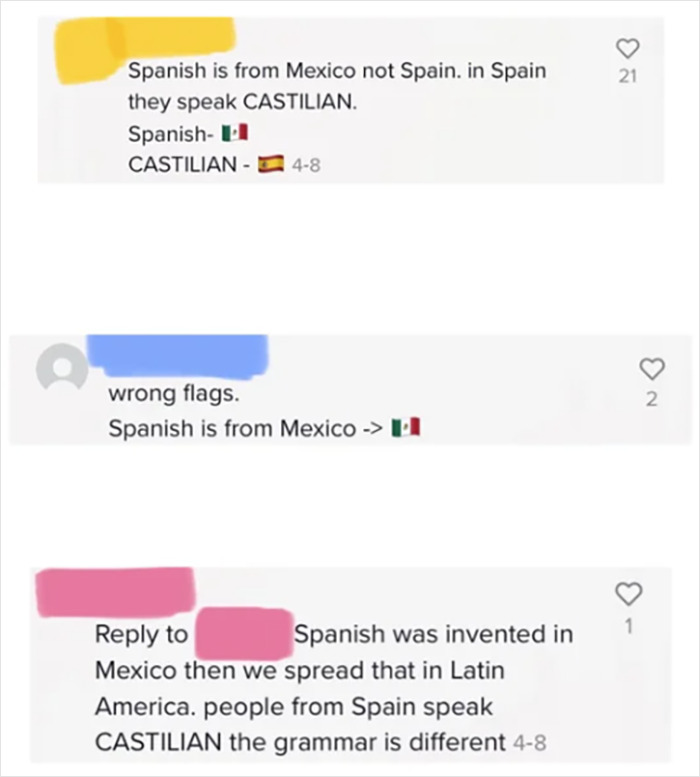This image appears to be a screenshot from an online forum with a white background and three distinct light gray text boxes. 

- **Top Gray Box:**
  - **Yellow Smear (Left Side):** Something obscured.
  - **Text (Below Smear):** "Spanish is from Mexico, not Spain. In Spain, they speak CASTELLANIAN."
  - **Icon/Flag:** A small image of the Mexican flag next to the word "Spanish."
  - **Icon/Flag:** A small image of Spain's flag next to the word "Castellanian."
  - **Number:** "4-8."
  - **Heart Icon:** On the right side, showing the number "21."

- **Middle Gray Box:**
  - **Circular Profile Image:** Anonymous profile with a dark gray background.
  - **Text:** "wrong flags" in lowercase.
  - **Text:** "Spanish is from Mexico >" followed by the Mexico flag image.
  - **Heart Icon:** On the right side, showing the number "2."

- **Bottom Gray Box:**
  - **Pink Smear:** Something obscured.
  - **Text:** "Reply to" followed by another pink smear.
  - **Text:** "Spanish was invented in Mexico then we spread that in Latin America. People from Spain speak CASTELLANIAN. The grammar is different. 4-8."
  - **Heart Icon:** Showing the number "1."

This detailed caption encapsulates the content and structure of the forum screenshot, highlighting critical elements such as the text content, icons, flags, colors, and user interactions.